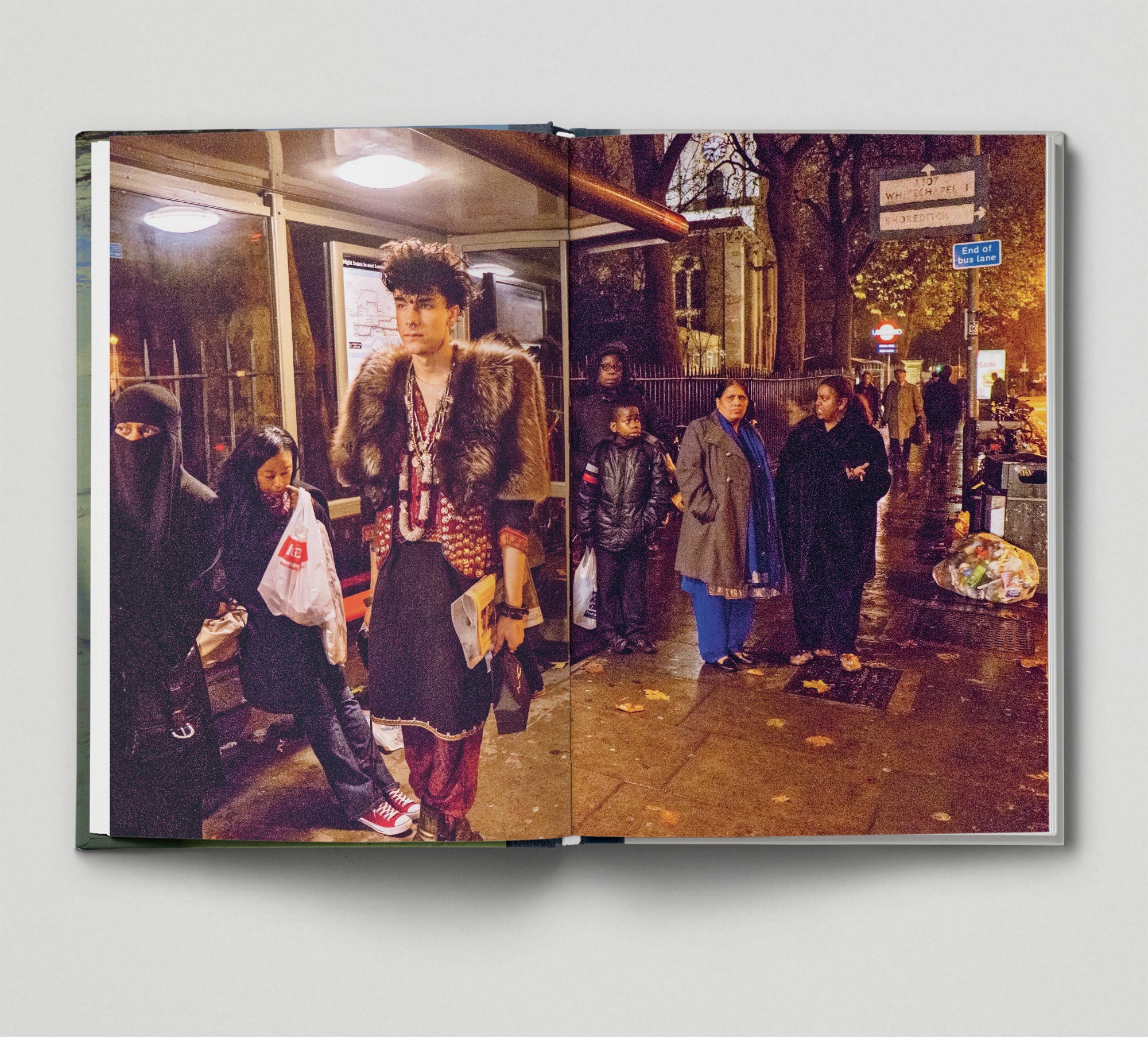The photograph depicts an open book with a green hard cover, resting on a light gray surface, opened to a double-page spread showing an urban scene at a bus stop. The center crease slightly interrupts the large image that spans both pages. The scene features a diverse group of people on a wet, leaf-strewn street. On the left side of the image, a woman with a black veil and a black purse with a large silver buckle stands next to a young girl holding a white plastic shopping bag, dressed in red shoes with white laces and bottoms, blue jeans, and a black jacket. To the right of them stands a man wearing a fur coat over a black skirt and red pants, with black shoes, short hair, and a necklace, holding a piece of paper. Further to the right, there is a black woman with a young black boy holding a white bag. Behind this group, several people with umbrellas can be seen crossing the street, adding to the scene's bustling atmosphere on what appears to be a dreary day. A blue street sign with white markings is visible, and the background shows a white sky. The ground features grates filled with fallen leaves and a bag of garbage next to a garbage can, completing the urban setting.